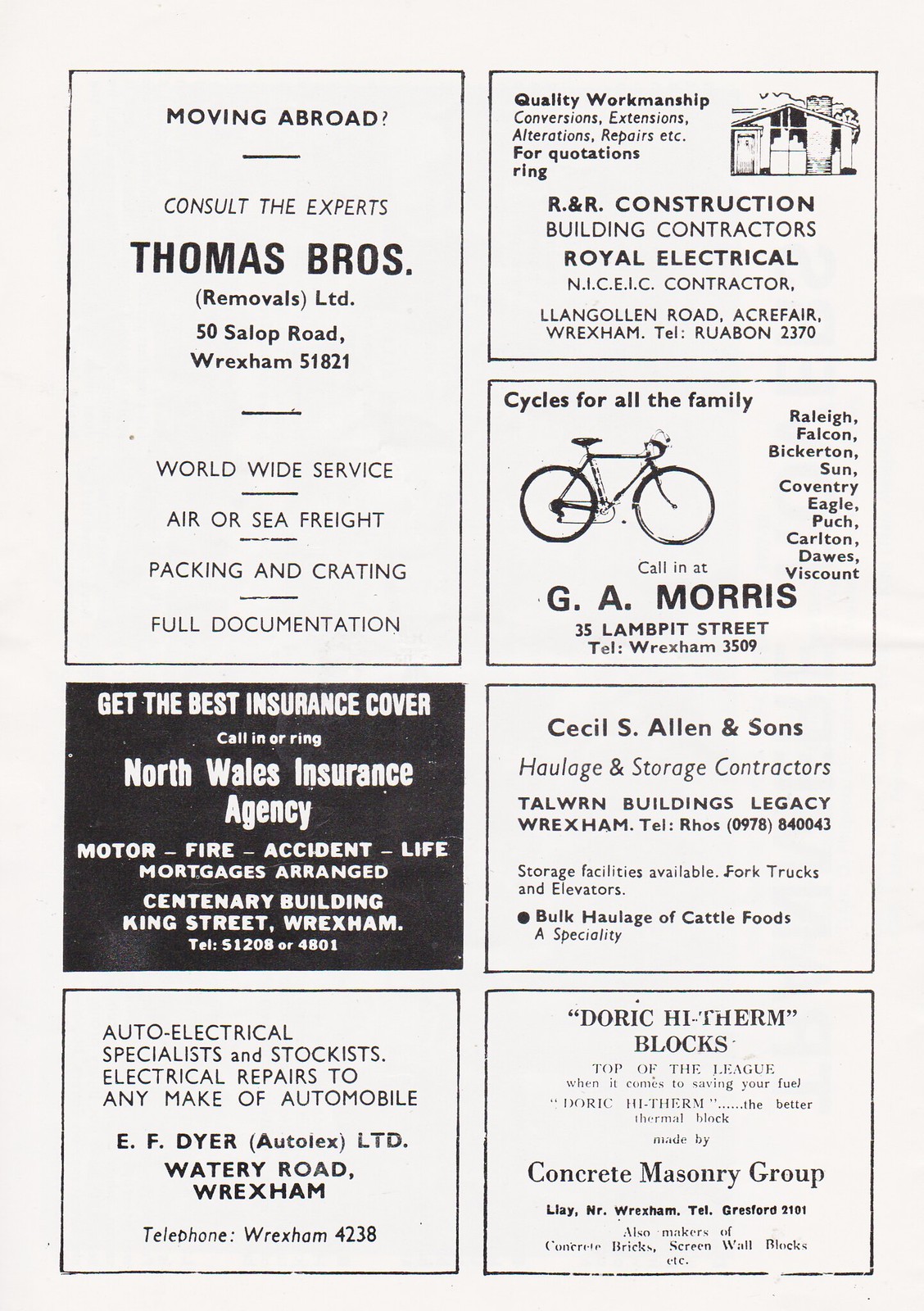This image captures a nostalgic advertisement page from an old magazine or newspaper, showcasing a variety of retro-style ads, all neatly enclosed in squares or rectangles. The layout is organized into two columns. In the first column:

1. **Thomas Brose:** This ad, with a white background and black text, announces services for individuals moving abroad, emphasizing "Worldwide Service, Air or Sea Freight, Packing and Crating, Full Documentation."
2. **North Wales Insurance Agency:** Featuring a black background with white text, it promotes insurance coverage for multiple needs including motor, fire, accident, and life, as well as mortgage arrangements.
3. **EF Dyer Auto Lex Limited:** This ad, also with a white background and black text, highlights their specialization in auto electrical repairs for any make of automobile.

In the second column:

1. **R&R Construction:** Displayed on a white background with black text, it showcases a stylized house and emphasizes their expertise as building contractors.
2. **G.A. Morris:** This advertisement, in a similar black-and-white theme, features a bicycle illustration and promotes cycling services or products.
3. **Cecil S. Allen and Sons:** This ad details their services in storage and college contracting.
4. **Doric High Therm Blocks by Concrete Masonry Group:** At the bottom, this ad on a white background with black text advertises construction materials.

All advertisements are tightly packed, creating a visually appealing tapestry of mid-20th-century commercial art.